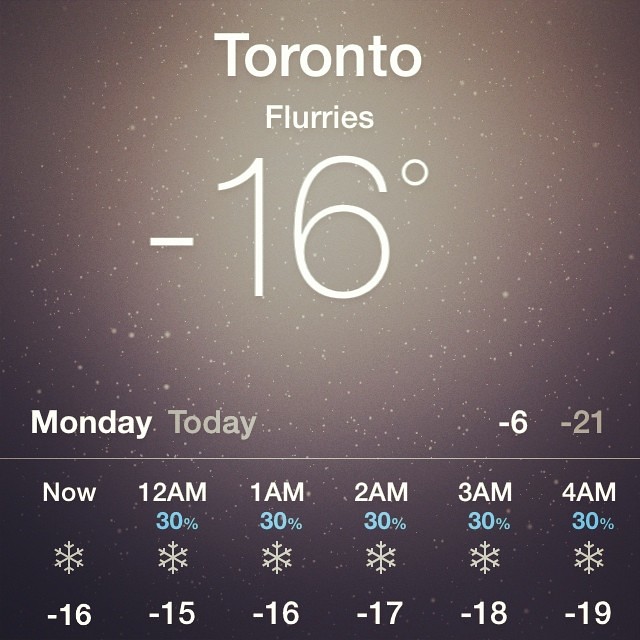The image depicts a weather information page for Toronto, indicated prominently by the large bold white letters in the header. Below the header, the current weather condition is described as flurries with the temperature prominently displayed as -16°C. The background of the image features a gray shade with white speckles, emblematic of falling snow. 

Underneath this, a detailed forecast for Monday is provided, segmented into six columns representing different times of the early morning. Each column features a small snowflake icon, reflecting the snowy conditions expected throughout the night. The columns are labeled with times starting from 12 a.m. to 4 a.m., with each time slot showing a 30% chance of snow. The associated temperatures for each hour are consistent with the frigid conditions, listing as follows: 

- 12 a.m.: -15°C
- 1 a.m.: -16°C
- 2 a.m.: -17°C
- 3 a.m.: -18°C
- 4 a.m.: -19°C 

This comprehensive hourly breakdown provides a clear depiction of the cold and snowy night anticipated in Toronto.